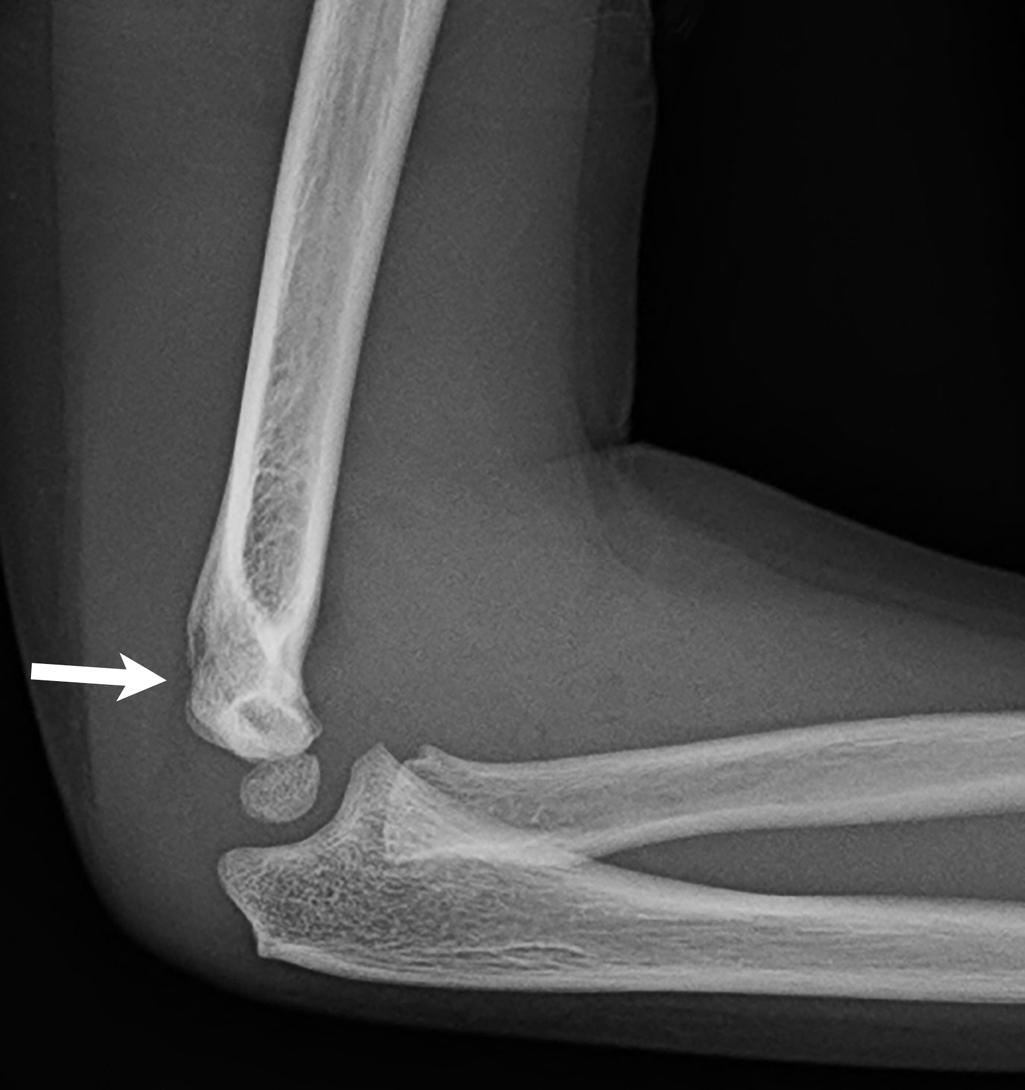This image depicts a black and white x-ray of a human arm bent at the elbow, captured in a close-up view. The background of the x-ray is solid black, providing a stark contrast to the grayscale hues of the arm's soft tissue and bones. The arm portion of the x-ray appears in dark gray, with the bones and joint highlighted in varying lighter shades. The x-ray reveals the bones of the forearm leading up to the elbow joint, where a white arrow points to a specific area of interest on the bone just before the joint.

There appears to be a small indentation or nick at the site marked by the arrow, suggesting a possible defect or fracture. The joint at the elbow includes a small section of bone resembling a spherical shape, indicative of the ball-and-socket structure. Another noteworthy feature is the split forearm bone structure, resembling a wishbone, extending towards the bottom left of the image. The bones display striations and diverse textures, with darker centers and lighter outlines, enhancing the detail of the skeletal structure visible in this high-contrast x-ray.